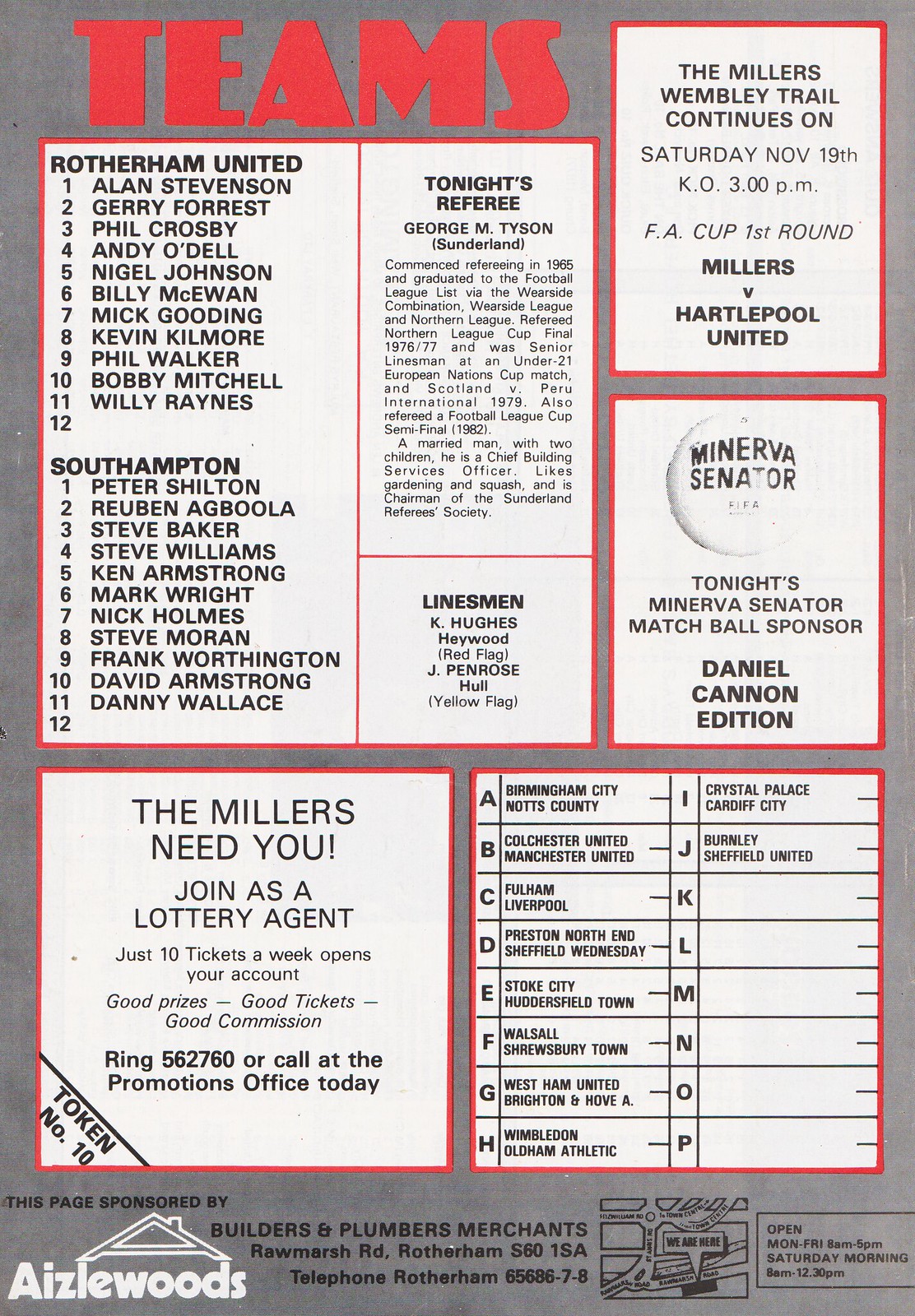The image is a promotional page, featuring several white rectangles with red borders and various texts on a grey background. At the top, in large red capital letters, is the title "TEAMS." Below this, details of two soccer teams' rosters are listed: Rotherham United and Southampton, each with players numbered from one to eleven. The page also mentions tonight's referee, George M. Tyson, and linesman, Kay Hughes. 

To the right of the team lists, it states "The Millers Wembley trial continues on Saturday November 19th, kickoff 3 p.m., FA Cup first round: Millers vs. Hartlepool." Beneath this text, there is a black-lettered soccer ball graphic labeled "Minerva Senator" and information about the matchball sponsor, Daniel Cannon.

At the bottom of the page, a promotion reads, "The Millers need you to join as a lottery agent." In the bottom-left corner is a logo with the text "ESL Woods" and the description "Hazel Woods Builders and Plumbers Merchants in Rotherham." To the right of this logo, there are additional symbols and details about the company, including unclear imagery that is too difficult to identify.